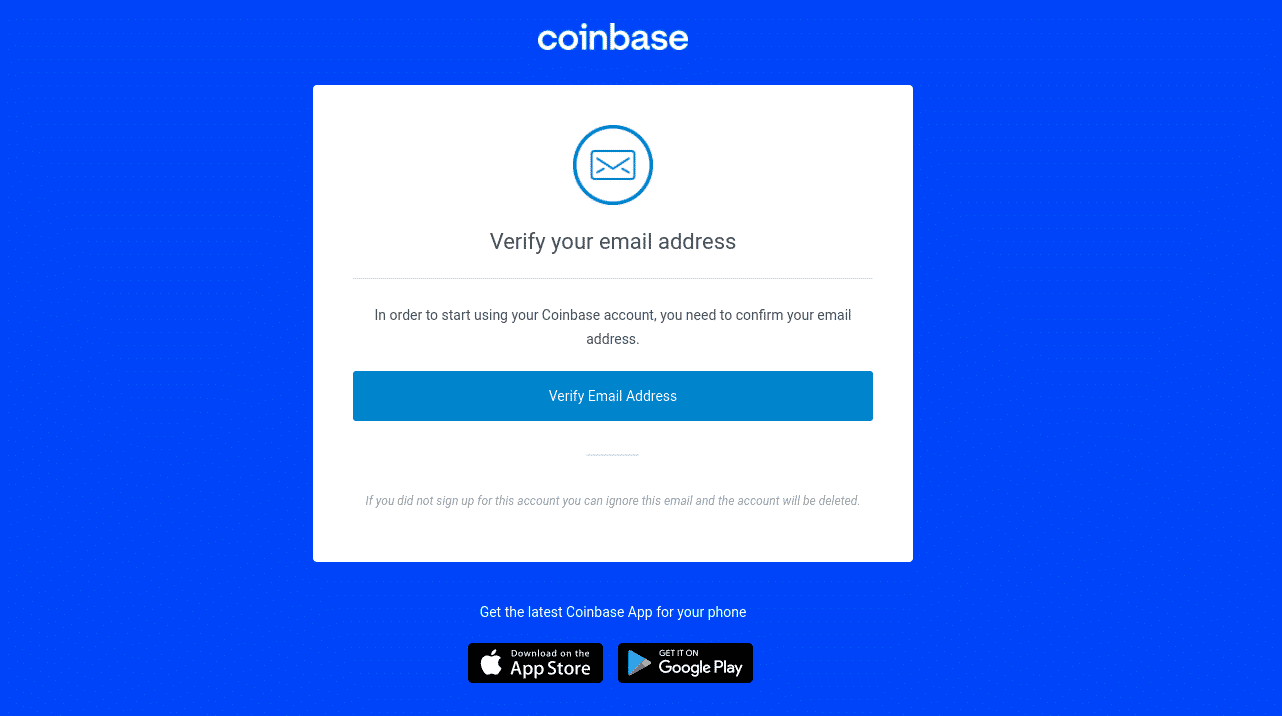The image is a rectangular notification from Coinbase, predominantly bright blue, with a longer horizontal dimension. At the top center, in white text, it reads "Coinbase." Below this, there is a white square featuring a blue-outlined circle with an envelope icon, also outlined in blue and filled with white. Beneath the icon, the text reads "Verify your email address" in black.

A horizontal line separates this section from the following explanatory text: "In order to start using your Coinbase account, you need to confirm your email address." 

Below this text is a long, teal blue button with "Verify Email Address" written on it in white. 

Underneath this button, a short line of text states: "If you did not sign up for this account, you can ignore this email and the account will be deleted."

Further down, the text against the blue background encourages: "Get the latest Coinbase app for your phone," written in white. This section includes icons for downloading the app from the Apple App Store and Google Play.

The primary colors used in the image are bright blue, teal blue, white, black, and gray. The purpose of this notification is to verify the user’s email address to prevent unauthorized account creation using someone else’s email.